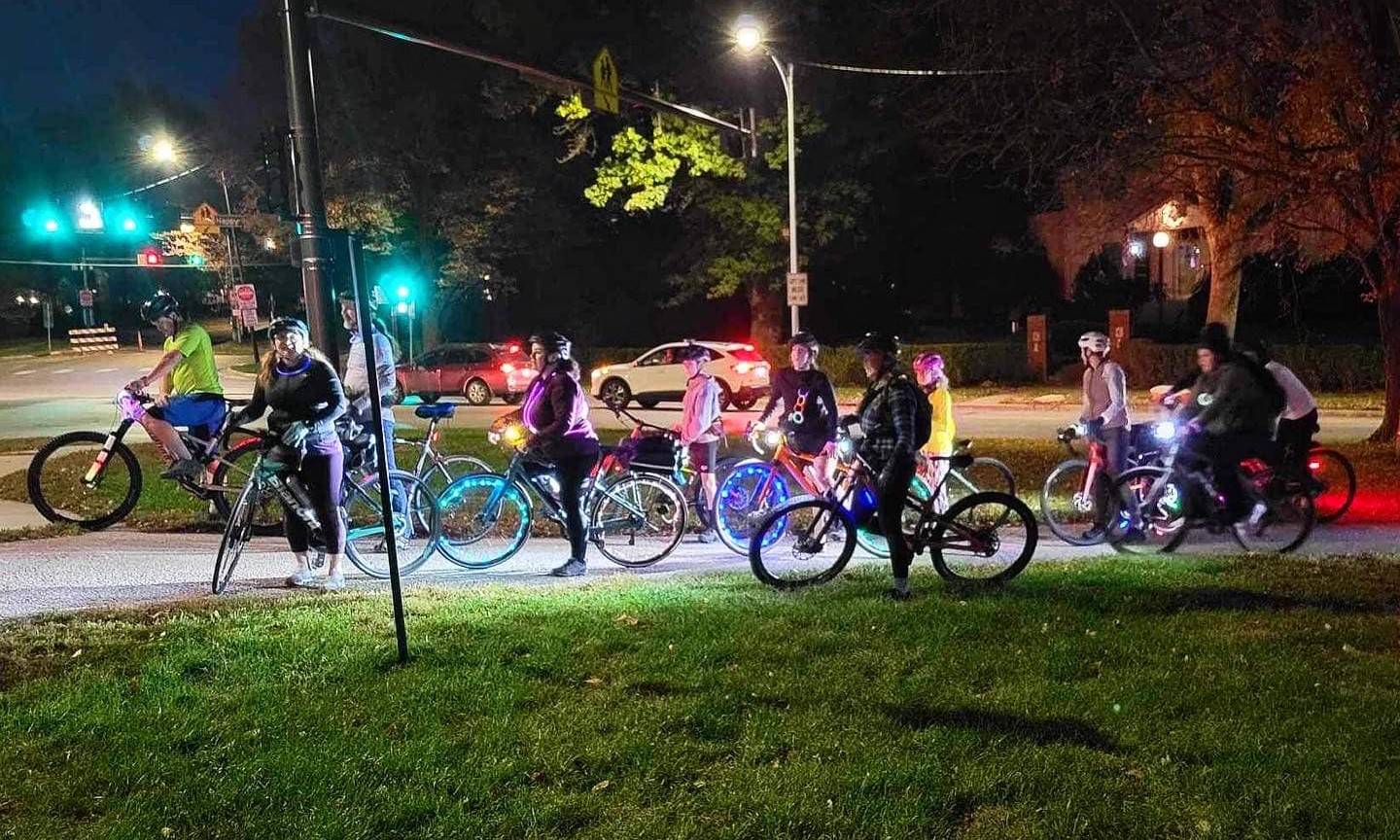This nighttime image captures a group bike ride with approximately 12 participants, composed of both children and adults, gathered on a sidewalk beside a concrete bicycle trail running from right to left. The cyclists, all equipped with helmets and bikes adorned with blue and white lights, are paused at a traffic intersection, where a mix of green grass, streetlights, and small residential houses lined with bushes and gates frame the scene. The cyclists, predominantly wearing long-sleeved shirts to brace against the cold, appear cheerful, some looking directly at the camera and smiling. The background reveals a street with two visible cars, one red and one white, amidst the dimly lit trees of the night, with green and red traffic lights casting an additional glow on the intersection. The atmosphere suggests a friendly group ride, temporarily halted at the signal, where the sense of community and shared enjoyment is palpable.